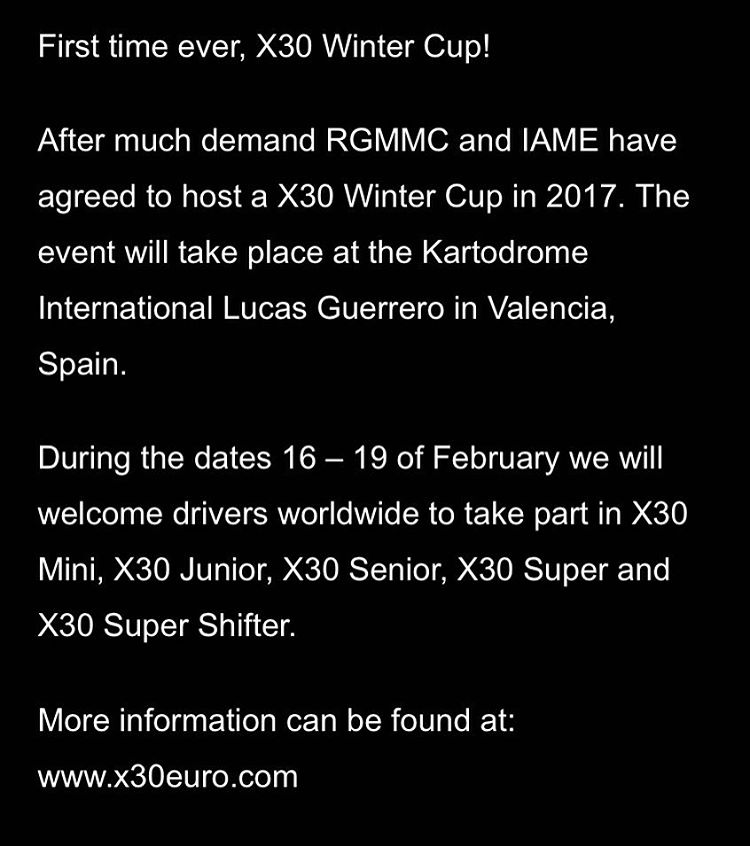The image features a simple and bold design with white sans serif text set against a completely black background, resembling a poster or advertisement. The prominent text announces, "First time ever X30 Winter Cup!" followed by detailed information about the event. After much demand, RGMMC and IAME have agreed to host the X30 Winter Cup in 2017. This exciting event will take place at the Cartodrome International Lucas Guerrero in Valencia, Spain, over the dates of February 16-19. During this period, drivers from around the world are invited to participate in various categories, including X30 Mini, X30 Junior, X30 Senior, X30 Super, and X30 Super Shifter. For further details, attendees are directed to visit the website www.x30euro.com. The text covers the entirety of the image, utilizing the stark contrast between black and white to draw attention to its content.